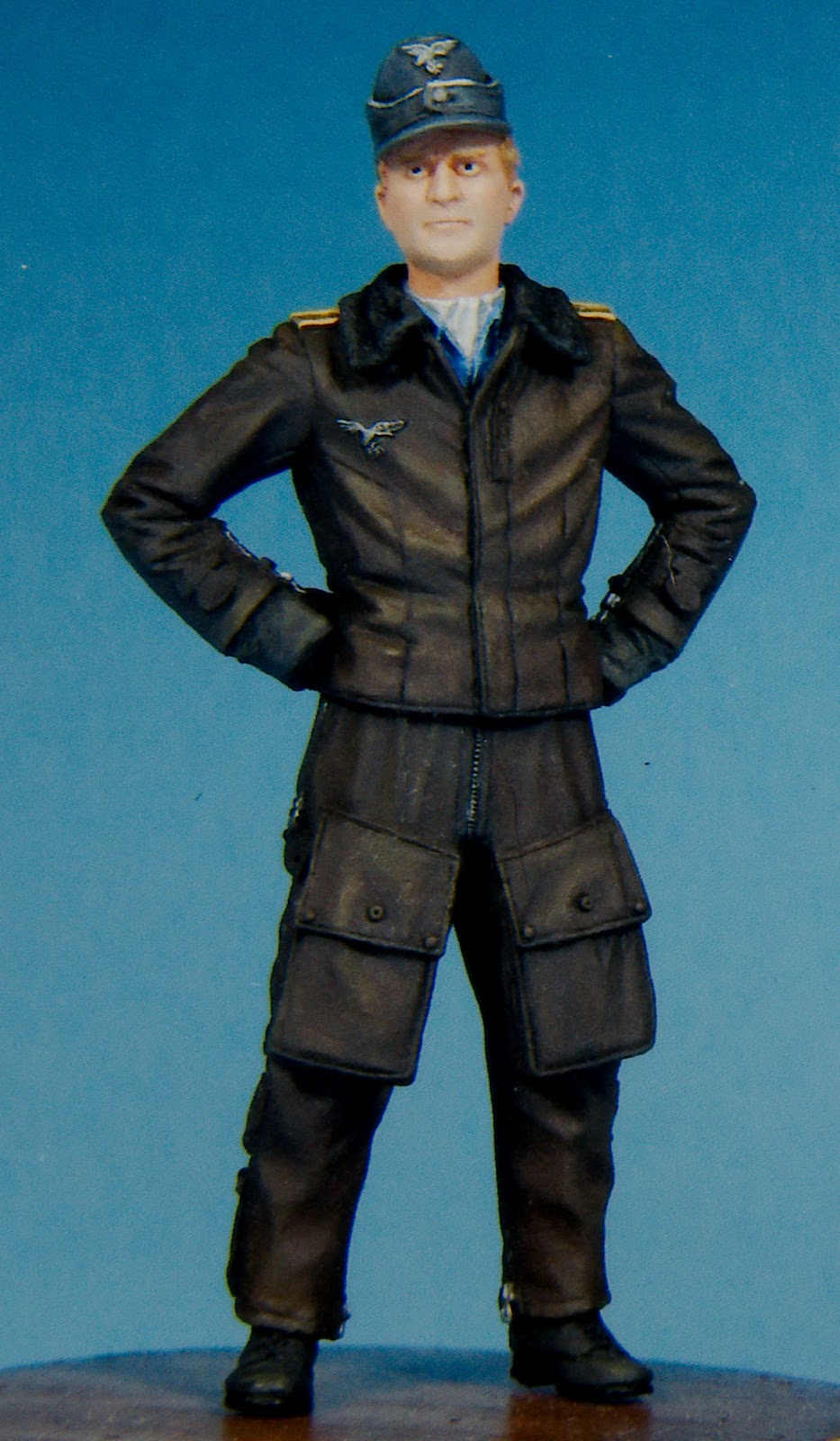The image depicts a grainy color illustration, reminiscent of early trading card art with suboptimal color reproduction. It features a Caucasian airman with blonde hair, standing against a blue background on a wooden surface. The airman is donning a blue cap adorned with wing symbols and is clad in a full leather flight uniform, composed of a dark leather flight jacket with an open collar, revealing a white shirt underneath. The jacket features an eagle flight logo on the right breast and long sleeves, complemented by black leather gloves. Gold horizontal bars adorn his shoulder epaulets. His hands are resting akimbo on his hips. The matching leather pants are equipped with rectangular long pouches, resembling old-fashioned mailbags, fastened with snap closures, positioned above each knee. Completing his attire are black combat boots. The overall aesthetic gives the impression of a historical fighter pilot, possibly a collectible figure or toy, evoking an Air Force theme.